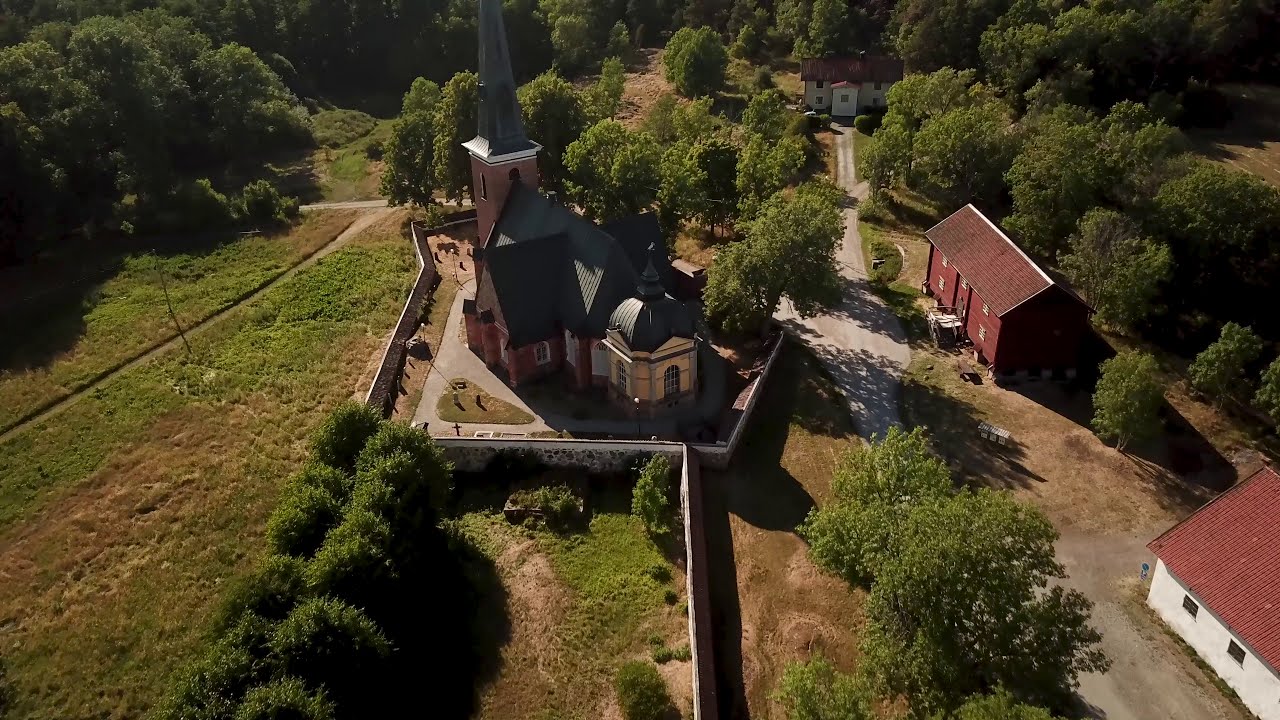This is an outdoor daytime overhead photo of a large, red brick home with a black roof, featuring a prominent tower on the right-hand side capped with a large triangular dome. To the right of the home, there is a white round structure with a black, pointy, triangular roof. The property is enclosed by a stone wall and surrounded by patches of grass, dirt fields, trees, and bushes. Shadows, cast by the sun from the upper left corner, stretch downward to the right-hand corner. A roadway runs alongside this brick home, curving off to the left. In the background, there’s another house, white with a brown roof, approximately two or three stories high, also encircled by dirt fields and green patches.